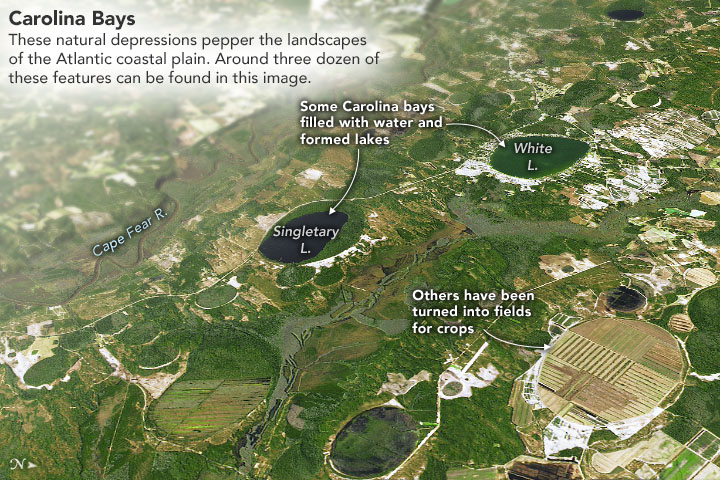An expansive aerial view reveals a lush, green landscape dotted with several buildings. The upper left corner features black print labeling the scene as "Carolina Bays," which are natural depressions scattered across the Atlantic coastal plain. In this image, approximately three dozen of these unique features are visible. To the left, the map indicates the presence of Cape Fear, while the lower right corner highlights an area where some of these depressions have been transformed into agricultural fields, evident from the orderly lines of crops. The upper right corner contains white text that identifies "White L" and "Singletary L," noting that some Carolina Bays have filled with water to form lakes.